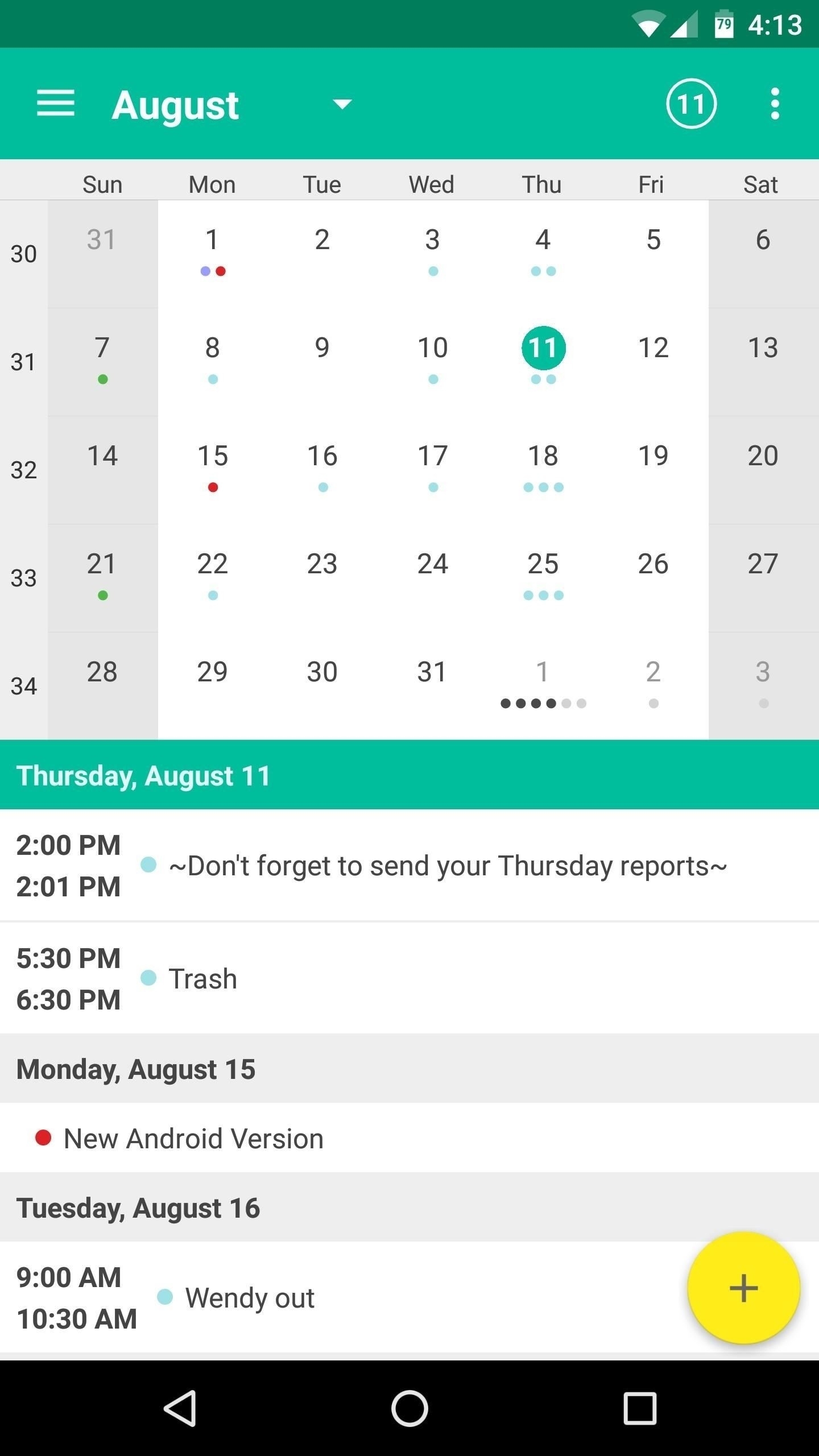This image is a screenshot from a smartphone displaying a calendar app. At the very top, the header is green, and on the right side, in white font, the time is shown as 4:13, with the battery level at 79%. Below this, there is a calendar with the header graphic in an aquamarine green color. On the left side of the header, the month "August" is written in white font, next to three horizontal lines that indicate a clickable menu.

The calendar displays the entire month of August. The days from Monday to Friday have a white background, while Saturday and Sunday have a very light gray background. Thursday, the 11th, is highlighted with a solid circle in the same aquamarine green color as the header, and the number 11 is written in white.

At the very bottom of the calendar, there is a green strip extending from left to right with "Thursday, August 11th" written in white font. Beneath this strip, against a white background, there is a list of activities for the day. Specifically, at 2:00 p.m., there is a reminder that says, "Don't forget to send your Thursday reports."